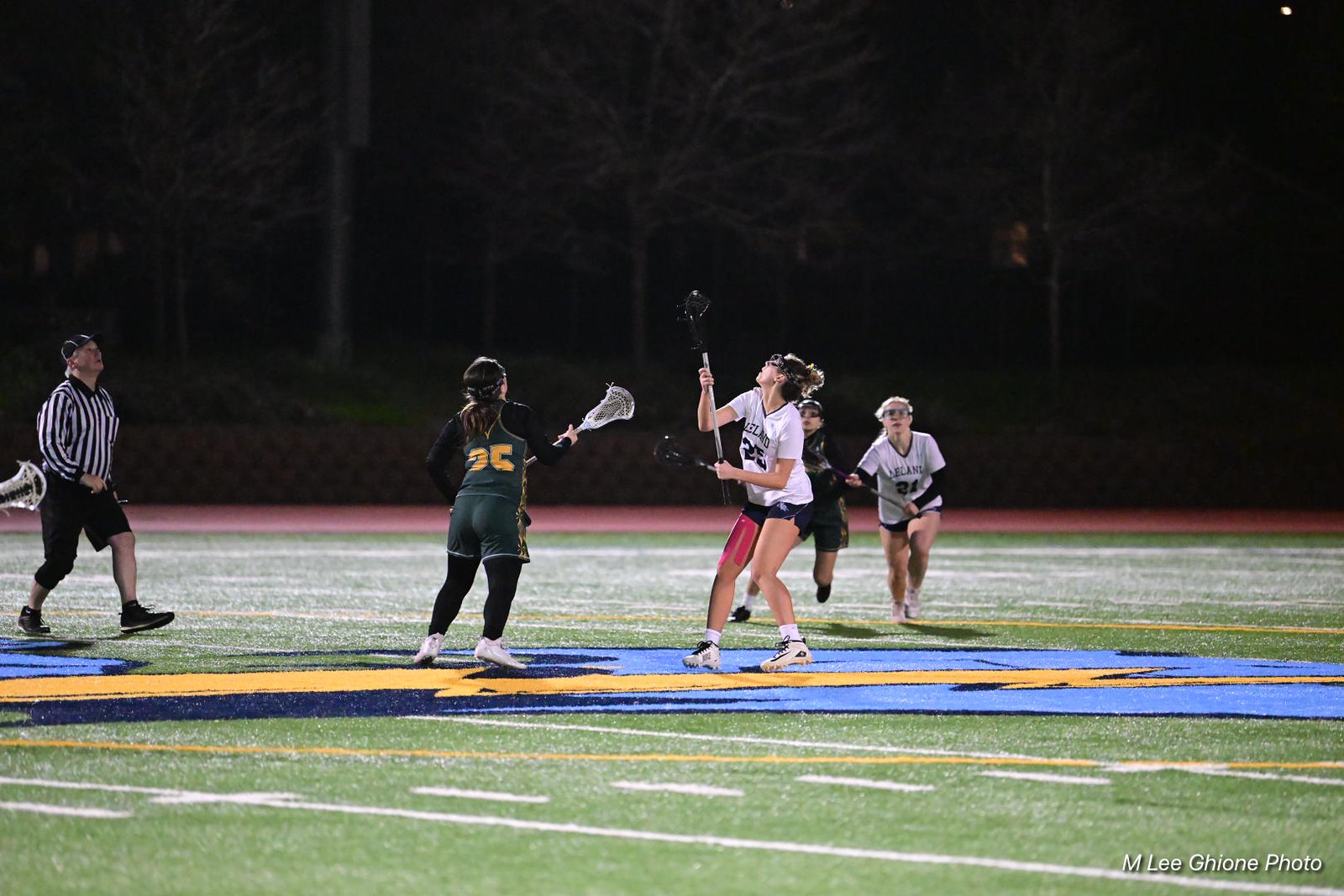This is a nighttime outdoor image of a high school lacrosse match on a green astroturf field, illuminated by the dark sky above. In the center, the main focus is on two female players vying for possession of a lacrosse ball. The player on the left is dressed in a green and yellow team uniform over black leggings, and she is adorned with white shoes and a headband. Her opponent, wearing a white shirt and blue shorts, has pink or red kinesiology tape visible and is also sporting white shoes. Both players are intently focused, their lacrosse sticks poised in the air. 

In the background, two more girls, one in green/yellow and the other in white/dark shorts, are running towards the middle to join the play. To the far left stands a referee, clad in a black and white striped shirt, black shorts, black knee brace, and black shoes, complete with a referee's cap. The backdrop features dark-colored trees, reinforcing the nighttime setting. The scene is set on a professional-looking field, marked by a red running track that borders the football field's edge and a large, indistinct blue and yellow logo at its center. The photo is credited to Emily Gion, as indicated in the bottom right corner.